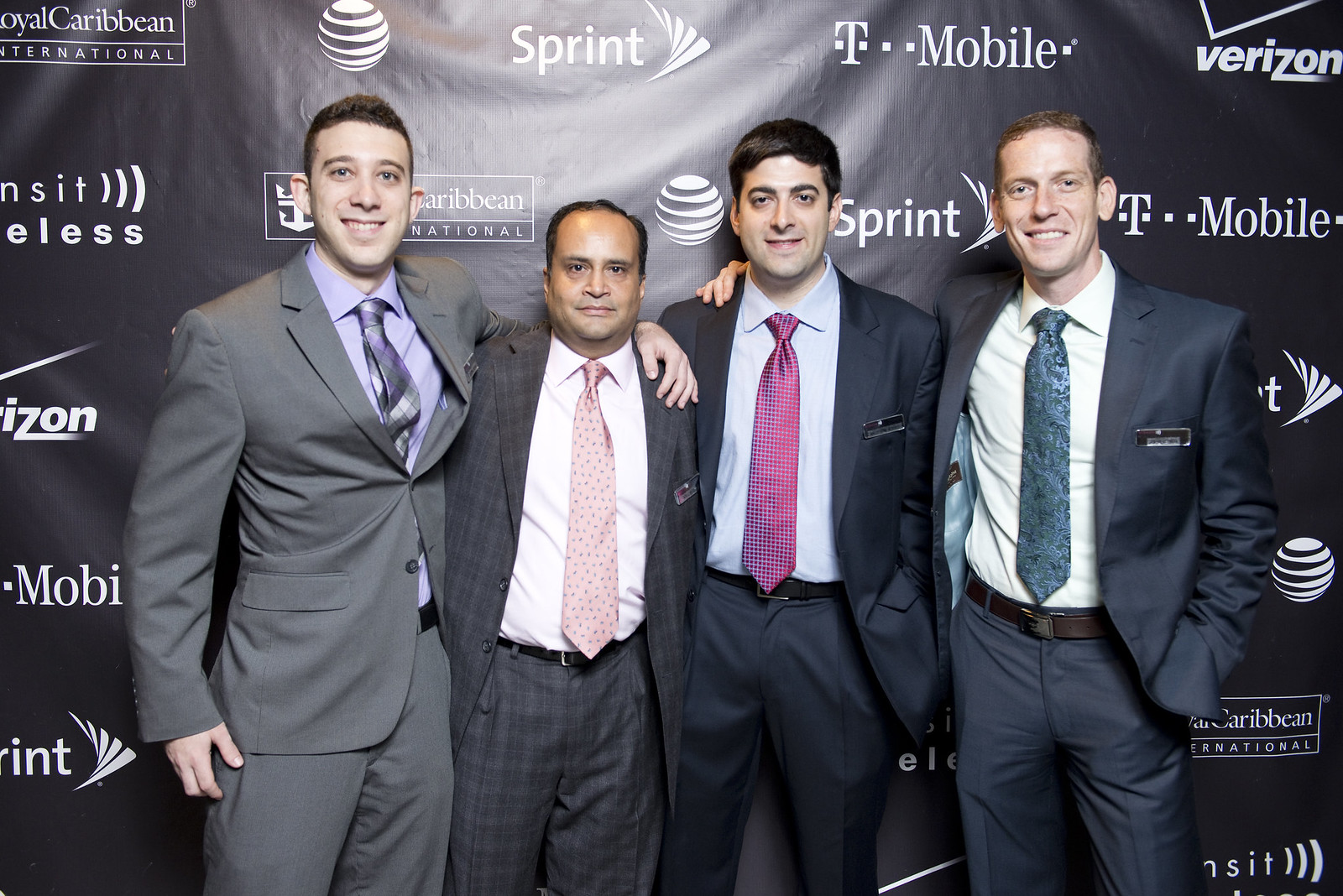In this image, four businessmen are posing together at a sponsored event, standing arm in arm and smiling for the camera. They are positioned in front of a black background decorated with white logos of various corporate sponsors such as Sprint, T-Mobile, AT&T, Verizon, and Royal Caribbean International. The men are dressed in business suits with ties in an array of colors: one wears a gray suit and pants with a purple shirt and tie, likely incorporating gray tones; another, possibly of Middle Eastern or Indian descent, is shorter with black hair, and wears a black suit with a white shirt and pink tie. A third man, who could be white or Hispanic, has black hair and is dressed in a blue suit with a blue undershirt and a red-and-blue tie. The fourth man, who is white with brown hair, is clad in a blue suit with a white shirt and blue tie. They are all evidently enjoying the event, comfortably standing shoulder to shoulder.